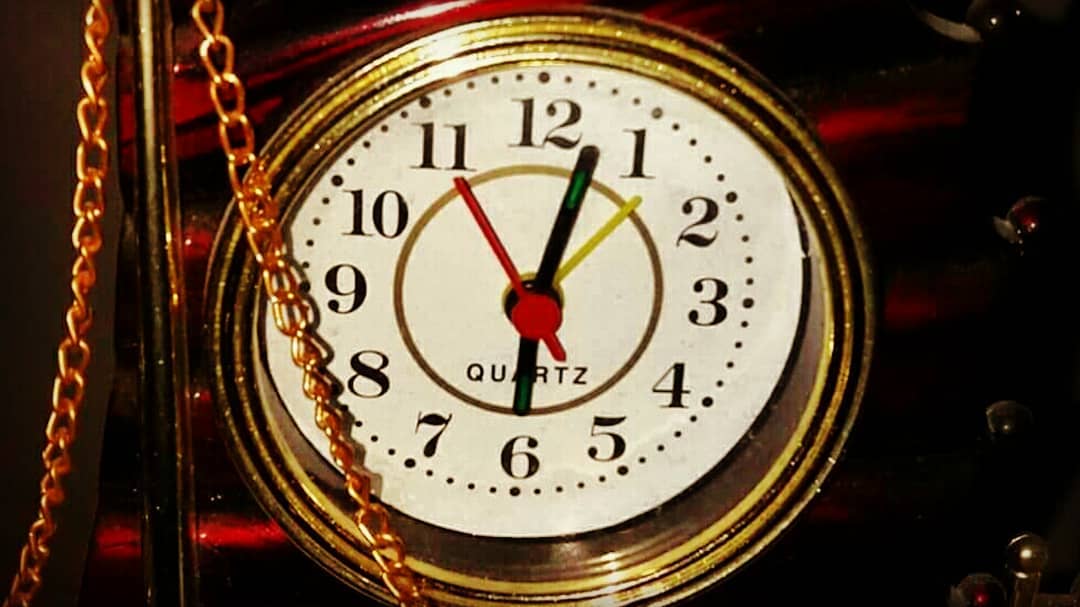The image depicts a meticulously designed clock with a striking gold frame, embellished with multiple beveled edges. Centrally positioned, the circular clock contrasts beautifully against a deep cherry red background, which appears to have a reflective, metallic sheen. Dominating the left side of the image is a vertical golden rod that extends from the bottom to the top, adorned with a luxurious golden chain that loops up the left side, crosses over the rod, and descends down the right side. The clock face itself is a pristine white, featuring bold black Arabic numerals. Intriguingly, the clock's hands are designed in red, black, and yellow, yet they are of nearly indistinguishable length, making it challenging to discern the exact time. Beneath the center where the hands converge, the word "quartz" is elegantly inscribed, indicating the clock's mechanism.